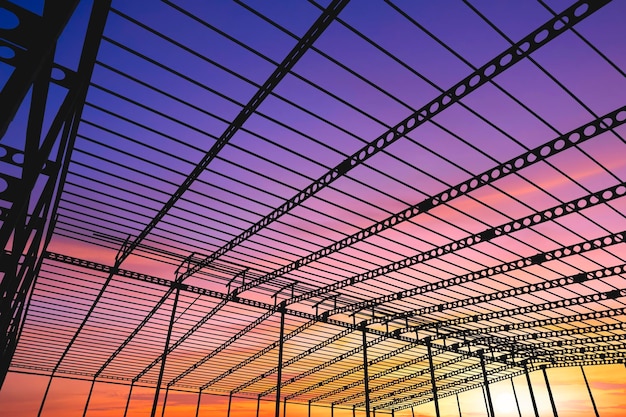The image captures a low-angle view of an incomplete metal structure, resembling a building under construction. The roof is an open framework of I-beams and metal rods arranged in a grid-like pattern, with the crisscrossing bars forming a partially transparent ceiling. The vertical supports and heavy stanchions are visible, holding up the intricate lattice of horizontal and diagonal bars. The background is dominated by a vibrant sunset that transitions from deep blues at the top to purples, pinks, and finally warm oranges and yellows near the horizon. The sunset illuminates the skeletal structure, casting uniform black shadows and creating a stark, yet beautiful contrast against the colorful sky.